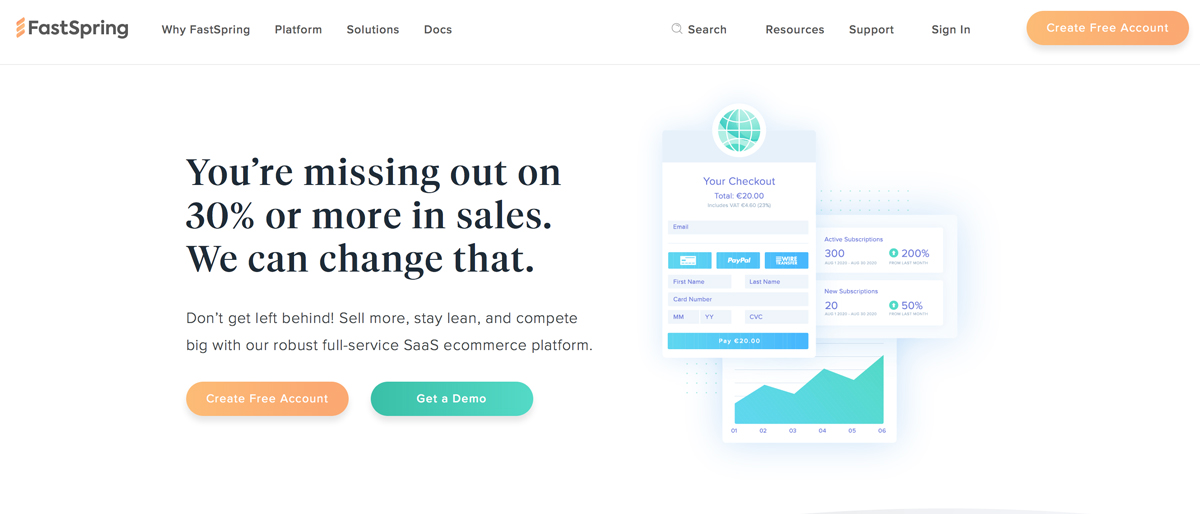This image is a screenshot of a website page. In the top left corner, the FastSpring logo is prominently displayed, featuring three diagonal orange lines to the left of the text. Moving right along the top navigation bar, options include "Why FastSpring," "Platform," "Solutions," "Docs," and towards the far right, an orange button with white text that reads "Create Free Account." Next to this button are links for "Sign In," "Support," "Resources," and a search icon represented by a gray magnifying glass.

Centered on the page is a large headline in bold black text stating, "You're missing out on 30% or more in sales. We could change that." Directly beneath it, a subheading reads, "Don't get left behind. Sell more, stay lean, and compete big with our robust full-service SaaS eCommerce platform." Below this text, two buttons are present: an orange button labeled "Create Free Account" and a green button labeled "Get a Demo."

To the right of this information is a graphic of a green globe encircled by a white ring, followed below by three images showcasing the website's interface. The bottom image features a green line graph displaying percentages and numbers, indicative of sales data. Above that is another graphic illustrating various credit card information input fields in different blue boxes, with text indicating a checkout total of 20 euros.